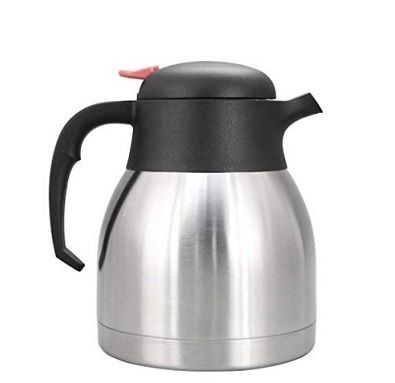This image showcases a retail product clearly presented against a clean, white background, typical for product displays. The product is an insulated carafe, characterized by its short, squat, and round design. The carafe features a stainless steel body for thermal insulation and a black plastic top, which includes a handle and a pour spout. The handle, designed for ergonomic use, does not extend all the way to the silver base of the carafe, ensuring a sleek profile. Notably, there is a small red lever on top of the lid, precisely positioned where the thumb would naturally rest, allowing for easy operation to open the lid. The black plastic portion, which consists of the pour spout and handle, appears as a single piece, and the top third of this plastic section can be twisted off to fill the carafe. Commonly seen in places like coffee bars or restaurants, this carafe is typically used for serving milk, creamer, or coffee, and is designed to maintain the temperature of its contents over extended periods.